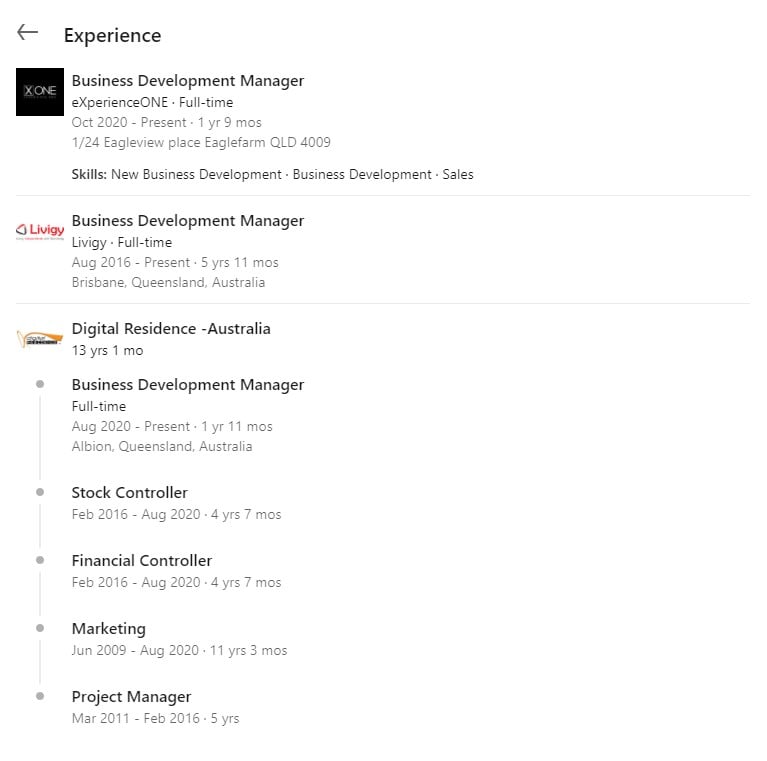The image features a white background with black text. At the top left, it reads "Experience" accompanied by a black button to its left. Below this header, the following detailed professional experiences are listed:

1. **Business Development Manager (Eagle View)**
   - **Employment Type:** Full-time
   - **Duration:** October 2020 - Present (1 year 9 months)
   - **Location:** 1 of 24 Eagle View Place, Eagle Farm, QLD 4009, Australia
   - **Skills:** New Business Development, Business Development, Sales
   - **Icon:** Black with white text "X 1"

2. **Business Development Manager (Niveki)**
   - **Employment Type:** Full-time
   - **Duration:** August 2016 - Present (5 years 11 months)
   - **Location:** Brisbane, Queensland, Australia
   - **Icon:** Red triangle with red and blue colors, featuring white text "Niveki"

3. **Business Development Manager (Digital Resident Australia)**
   - **Employment Type:** Full-time
   - **Duration:** August 2020 - Present (1 year 11 months)
   - **Location:** Albion, Queensland, Australia

4. **Stock Controller (Digital Resident Australia)**
   - **Employment Type:** Full-time
   - **Duration:** February 2016 - August 2020 (4 years 7 months)

5. **Financial Controller (Digital Resident Australia)**
   - **Employment Type:** Full-time
   - **Duration:** February 2016 - August 2020 (4 years 7 months)

6. **Marketing (Digital Resident Australia)**
   - **Employment Type:** Full-time
   - **Duration:** June 2009 - August 2020 (11 years 3 months)

7. **Project Manager (Digital Resident Australia)**
   - **Employment Type:** Full-time
   - **Duration:** March 2011 - February 2016 (5 years)

All experiences listed after "Digital Resident Australia" fall under the employment history with that specific company.